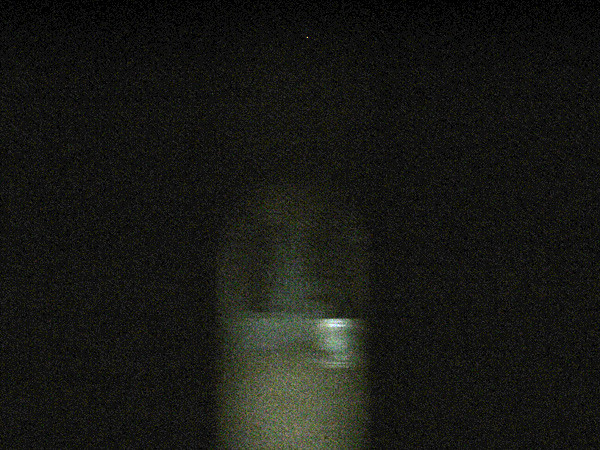The image is dark and grainy, suggesting it was taken under low light conditions, possibly outdoors at night or in a dimly lit room. The background is predominantly black, with a scattering of lighter pixels at the top, which might indicate stars, rain, or dust captured by a high ISO camera setting. In the center, a faintly illuminated rectangular structure with rounded edges at the top stands out. This structure has a light greenish hue at its upper section, transitioning to darker black and lightly colored portions below. The light source itself isn’t visible but casts a glow on this vertical structure, hinting at a distant origin, perhaps reflecting off a wall or similar flat surface. The image conveys a faint impression of a lighter sky above, reinforcing the outdoor night scene.